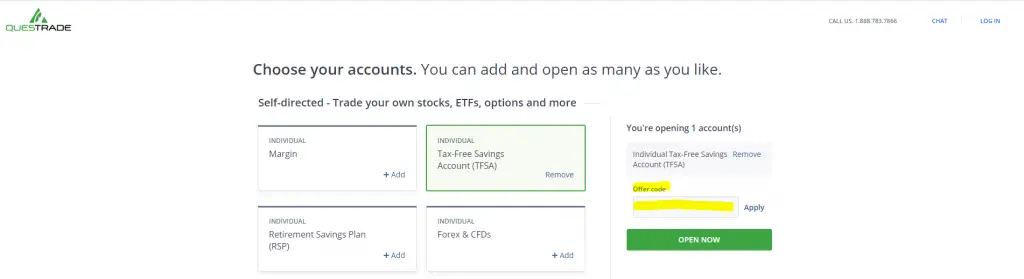The image is a screenshot from a Quest Trade platform, displaying an interface for choosing different types of accounts to open. The main title reads, "Choose Your Accounts," followed by an instruction indicating that users can "add and open as many as you like." Below this, it provides options for various types of accounts:

1. **Individual Margin**: Accompanied by a blue "plus" symbol indicating the option to add this account.
2. **Individual Tax-Free Savings Account (TFSA)**: This option is highlighted with a green outline and green background, denoting it is currently selected. There is also a "remove" option alongside it.
3. **Individual Retirement Savings Plan (RSP)**: With a blue "plus" symbol, suggesting it can be added.
4. **Individual Forex and CFDs**: Also featuring a blue "plus" symbol for addition.

On the right-hand side, there is a section confirming that the user is opening one account, specifically the "Individual Tax-Free Savings (TFSA)." It includes a "remove account" option and a field for applying an "offer code," with adjacent boxes highlighted in yellow. Further down, there is a noticeable green rectangle with white text that says "Open Now." The other three account options, which are not highlighted, have a white background with navy blue stripes running along the top edge of each rectangle.